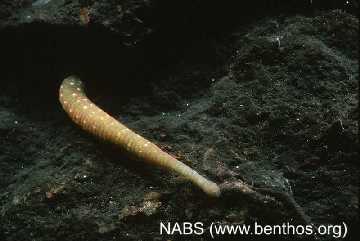This underwater photograph, taken near a coral reef or the ocean floor, presents a captivating scene of marine life. Dominating the image is a distinctive, elongated creature partially emerging from a dark hole in the rocky seabed located in the upper left corner. This creature, possibly an eel or worm, displays a striking pattern along its approximately 12-inch body—green with white spots and circular yellow stripes, transitioning to a grayish tip. The terrain features jagged rocks in hues of black, dark gray, and deep green, adding to the depth and complexity of the scene. In the lower right corner, the photograph is marked with the letters "N.A.B.S." and the website "www.benthos.org," indicating a connection to a marine studies organization. The mesmerizing interplay of colors and textures makes this underwater mystery both intriguing and visually compelling.